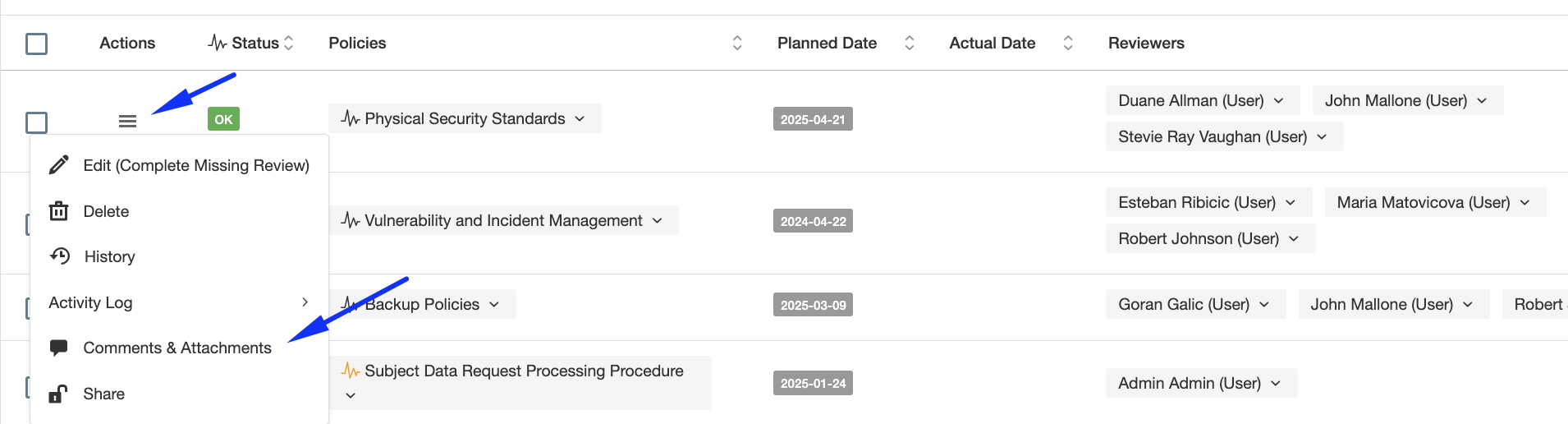The image features a detailed document layout, most likely created using a Microsoft Office tool such as Excel. The document appears to be a structured form or template aimed at managing a company's data processing procedures and security standards.

**Top Section:**
- Title: "Backup Policy, Subject Data Request Processing Procedure"
- Descriptors: The interface includes various menu options on the left such as "Edit," "Complete," "Missing Review," "Delete History," "Activity Log," "Comments and Attachments," and "Share."
 
**Columns and Headers:**
- Top Header Row: "Action Status Policies," "Plan Date," "Actual Date," and "Reviewers."

**Main Body:**
- Three main sections are detailed in rows from left to right:
  1. **Physical Security Standards:** 
     - Contains columns including "Date" and "Name."
     - Features names of multiple users.
  2. **Vulnerability Incident Management:** 
     - Similar structure with user names listed.
     - Example entry includes three names per row, with a potential fourth on incomplete rows.
  3. **Subject Data Request Processing Procedure:**
     - Noted for listing a single "Administration" name.

Overall, the document is a form intended for organizational use, detailing policies and procedures related to data requests, incident management, and physical security, complete with sections for user names and dates for tracking and review purposes.